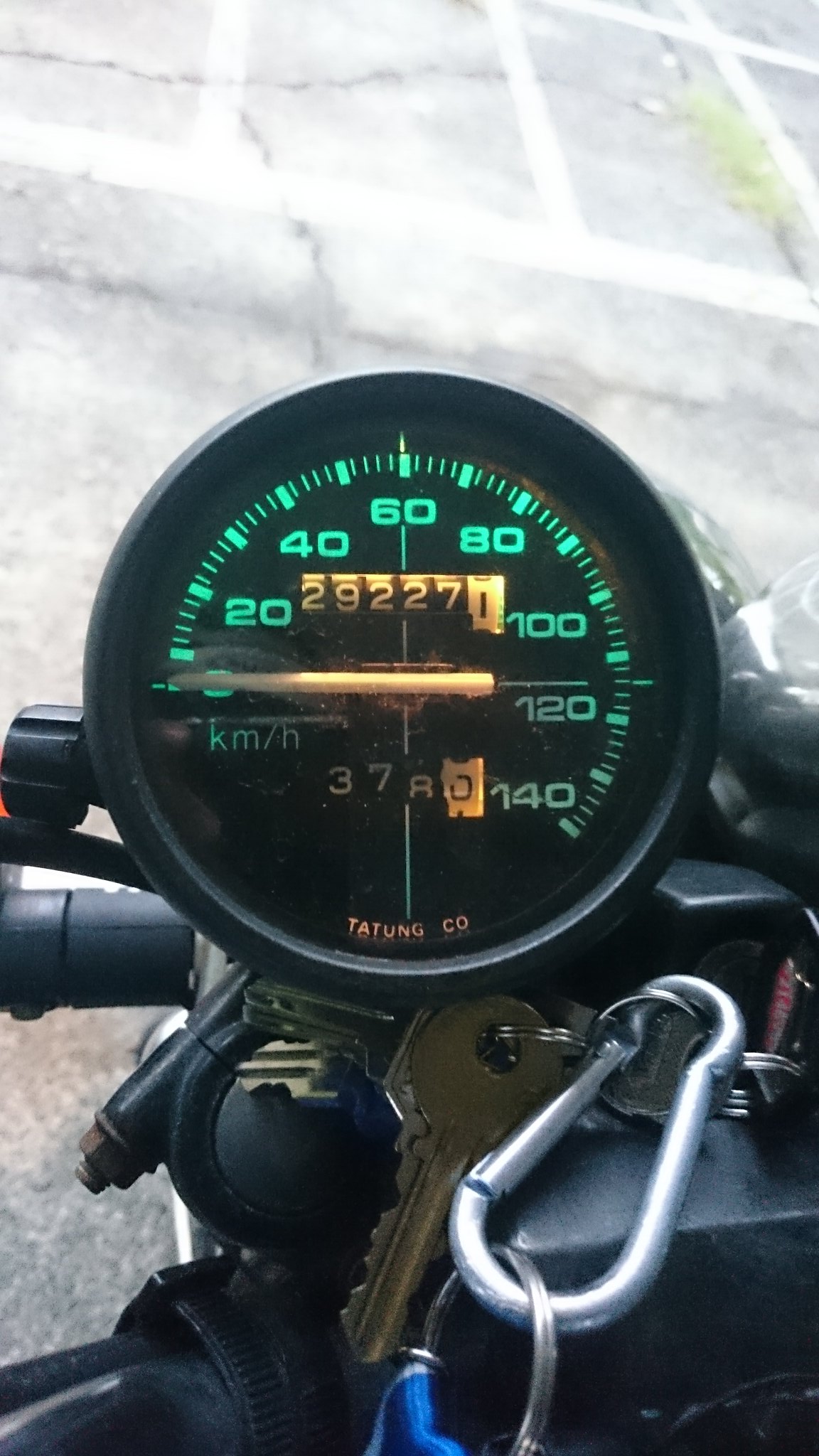The vertical image, approximately twice as tall as it is wide, prominently features a centrally-positioned gauge. This gauge, which resembles a speedometer, has a black rim with a matching black face. The numbers and dashes that line the gauge are backlit with a distinctive teal illumination, providing high visibility. At the center of the gauge, the odometer display is illuminated with a standard light, differing from the teal accents. Below this, the trip mileage indicator is clearly visible. Notably, the speedometer needle is white and positioned at zero, indicating the vehicle is at a standstill.

Attached to the upper left-hand side of a motorcycle or similar vehicle, the gauge is prominently displayed. Part of the black handlebar extends from behind and beneath the gauge. Just below the speedometer, there appears to be a keyring hook. The keyring is silver with a side-push mechanism and holds a loop of blue fabric alongside several gold keys. The motorcycle's dash, also black, is partially visible in the lower right-hand corner of the image, complementing the overall black aesthetic. The background appears to be a section of blacktop surface.